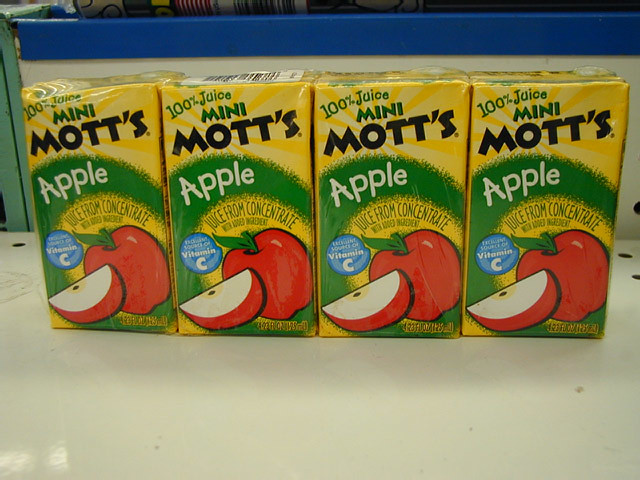This photo captures four yellow boxes of Mott's 100% Apple Juice Mini, neatly lined up side by side on a white countertop. The boxes are bundled together in a plastic wrapping and display vivid, consistent details. Each rectangular box features a prominent green circle in the center with 'Apple' written in white text. Above this, on the yellow background, 'Mott's' is stated in bold black text, and above that, it says '100% Juice Mini' in black letters. A red cartoon apple with a green stem and an adjoining apple slice is located at the bottom right of each box. Nearby, a blue circle announces 'Vitamin C' in white font. The package also notes 'Juice from Concentrate' near the apple imagery. The background includes a white wall with a blue border at the top and a small glimpse of a green wall to the left.